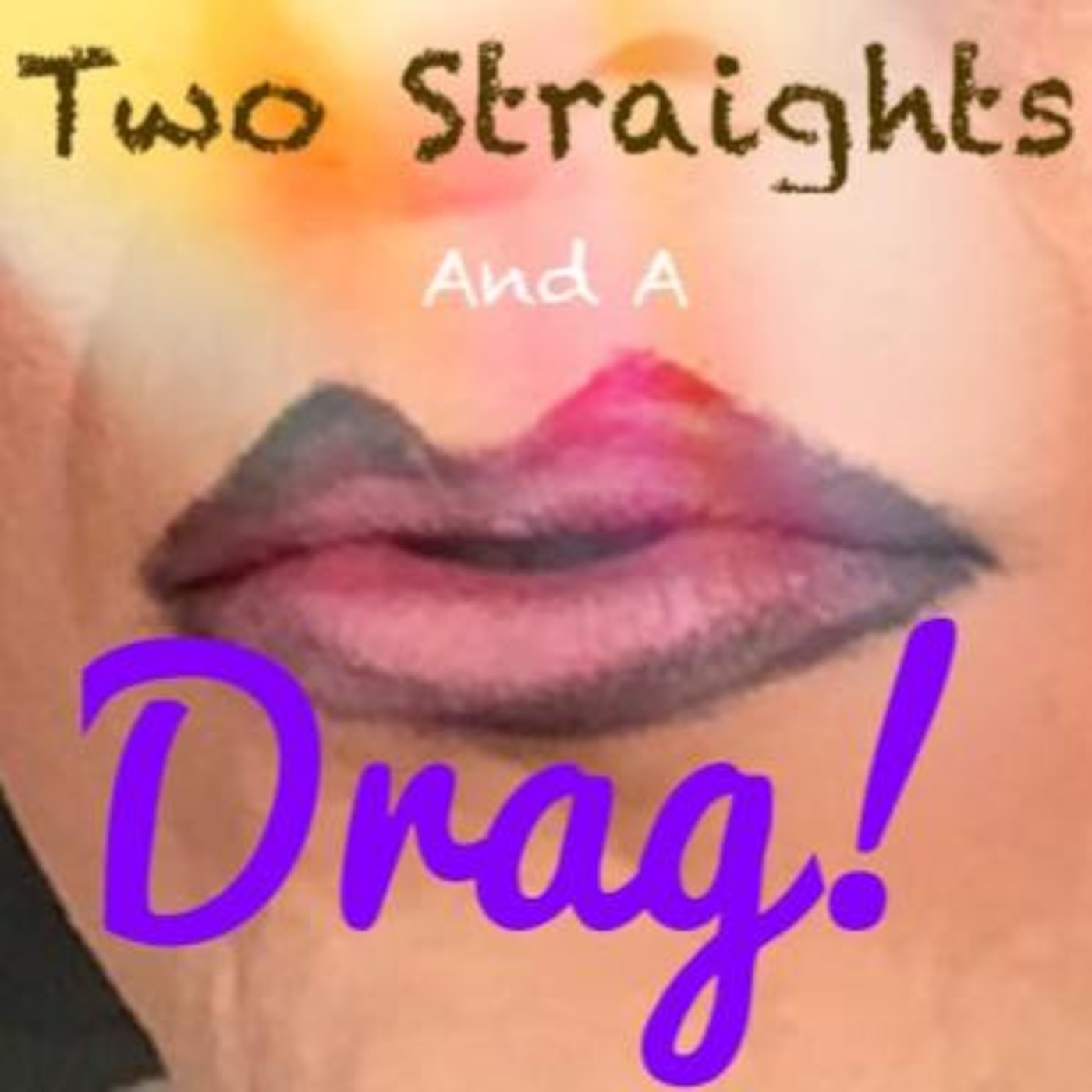The image is a low-quality, square advertisement for a show or video blog, with the face of a person—likely a Caucasian woman—almost entirely filling the frame. The focus is on her lips, which are positioned at the center and painted with a pinkish-red lipstick that fades to black. Above the lips, you can see the tip of her nose and the sides of her cheeks, but the details are somewhat obscured by the poor image quality. The background is a solid black color. 

The text in the image is formatted distinctively: "two straights" is written in large brown crayon-style text at the top of the frame, with "and a" in smaller white letters just below it. At the bottom, directly beneath the lips, "drag!" is displayed in large, cursive purple script. The overall impression is of an eye-catching, bold design intended to draw attention to the show's title.